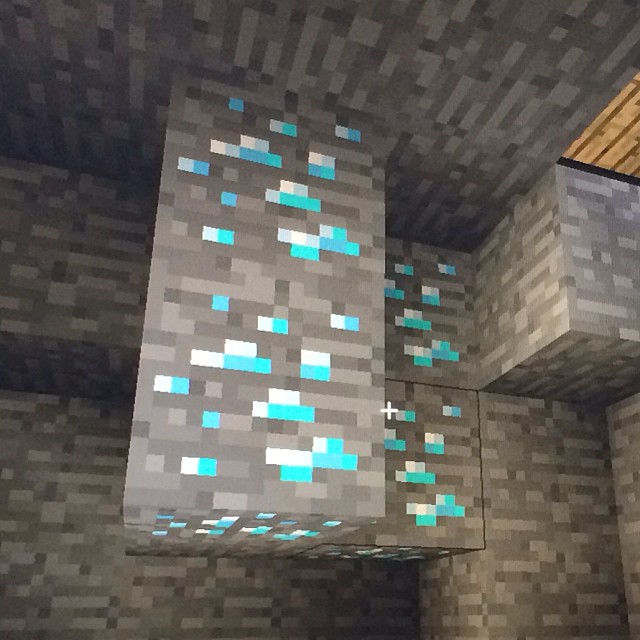The image is a partial screenshot from the game Minecraft, characterized by its highly pixelated, blocky aesthetics typical of the game. The screenshot captures an indoor area that appears to be constructed with various shades of brown, gray, and black blocks, indicating a likely underground setting. Prominently, there is a white crosshair offset from the center, suggesting it's not a full-screen capture. The blocks in the image exhibit a mix of plain brown and those with additional colors and patterns, including variations of white, green, blue, light blue, and turquoise, likely representing different materials or minerals within the game. Some blocks form a 3D structure, protruding towards the viewer, while others, notably three from the ceiling, incorporate a blend of dark gray, light gray, and colored mineral features. The right side of the image hints at the beginning of a brown rectangular bridge, contributing to the intricate layout of the scene.